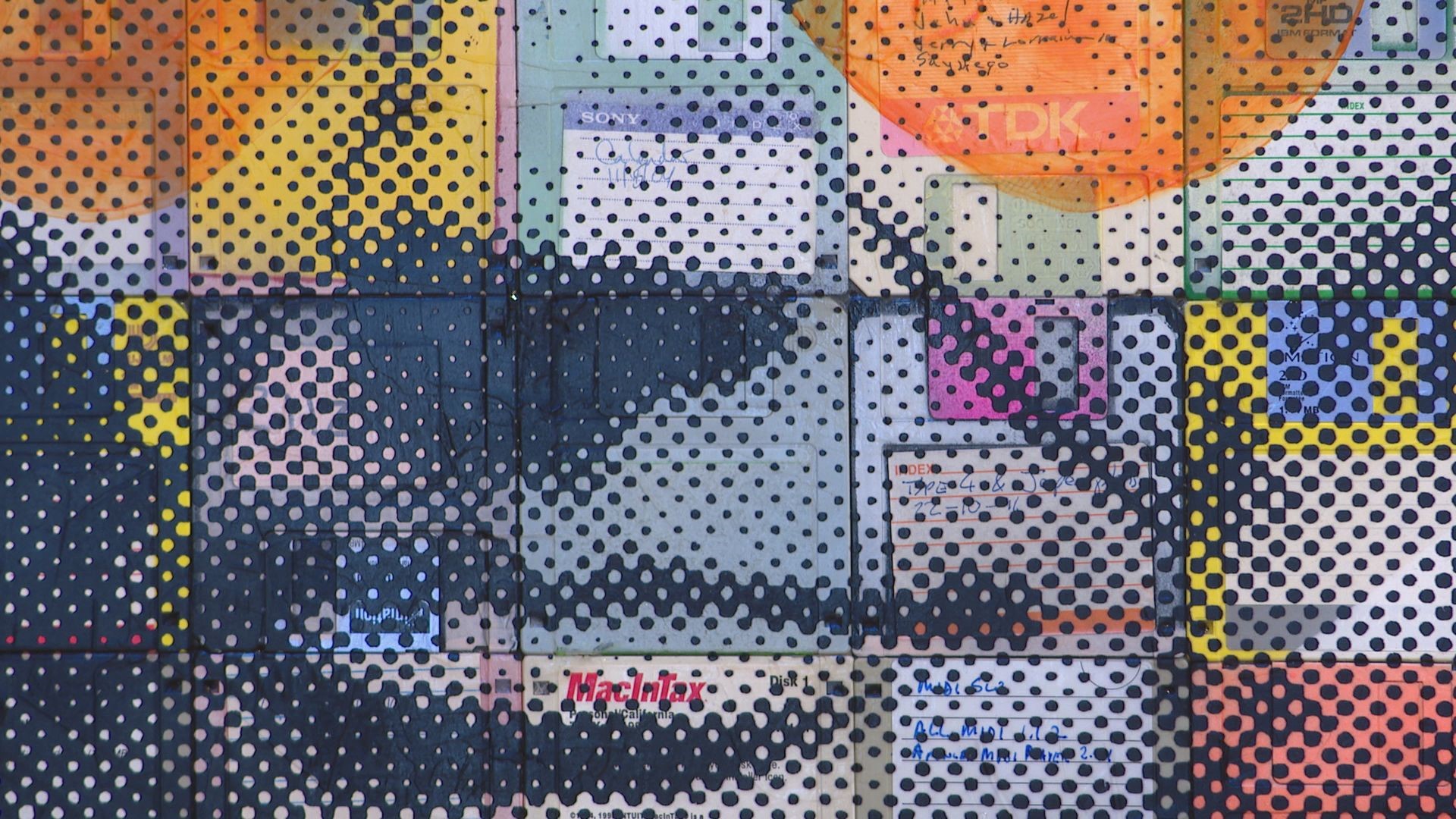This vibrant and nostalgic image is a detailed artistic print composed of various squares and quadrants, each featuring a unique design. The foundation of each square appears to be a retro mini-disc, with colors ranging from blue and white to purple, yellow, and orange, creating a diverse palette. The squares are overlaid with dots, some more concentrated than others, contributing to the overall sense of a pixelated mosaic. Among these dots, viewers can discern the stylized features of a woman’s mouth and nose, primarily depicted in dark and light blue. The print incorporates elements of pop art and cartoon styles, reminiscent of the 1980s nostalgia, complete with logos such as TDK and possibly Sony and Memorex, evoking memories of lo-fi VHS tapes and cassette culture from that era. The combination of color, dots, and retro imagery creates a visually compelling homage to the past, blending artistic creativity with technological nostalgia.